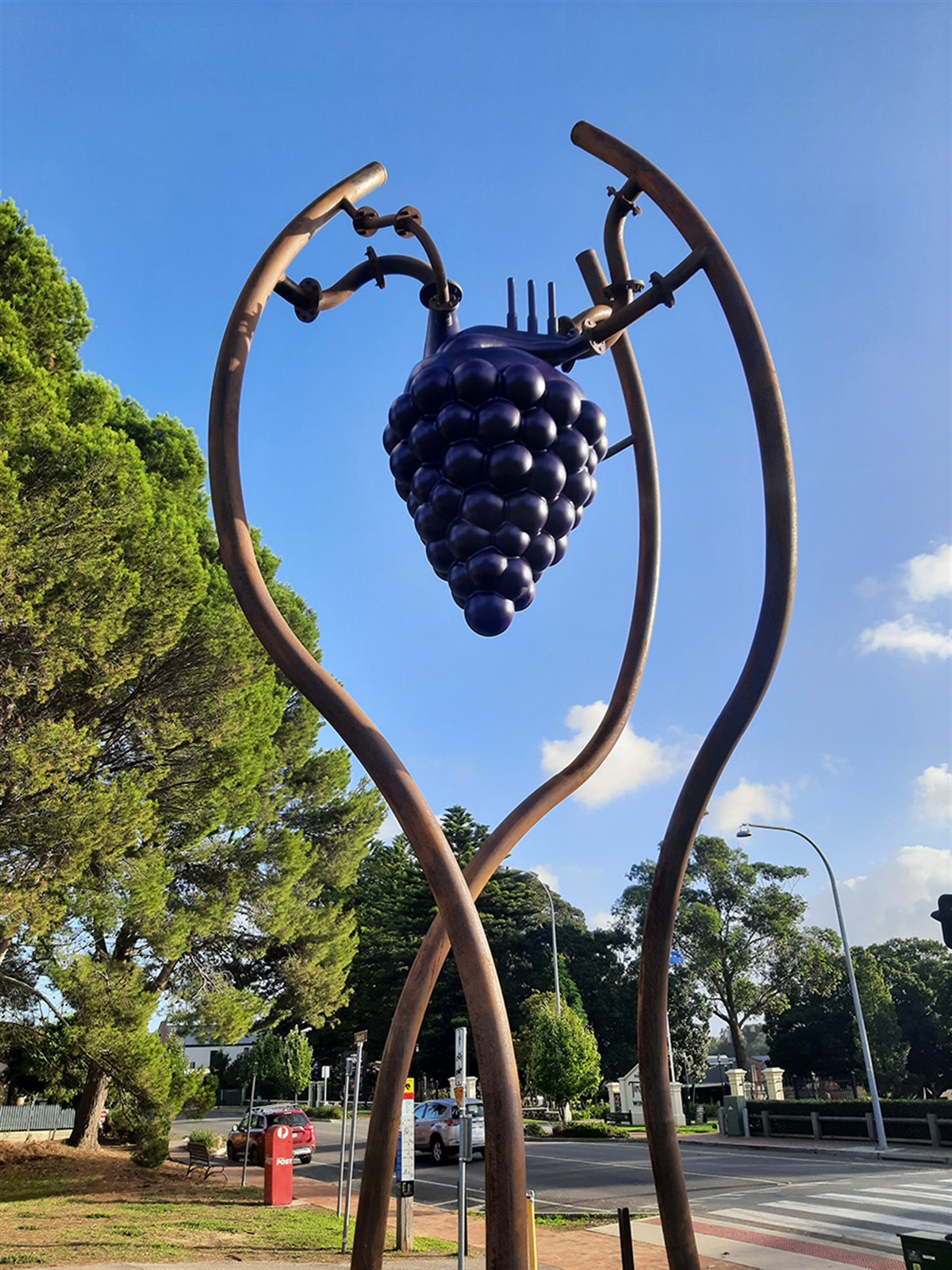The photo depicts an outdoor scene, likely in a park area adjacent to a roadside, featuring a prominent metal sculpture. The sculpture consists of three bronze-colored, curvy stems that extend from the ground and converge at the top, where they support a cluster of purple grapes, adding a striking visual element. Surrounding the sculpture, the scene includes lush greenery with a notable large tree on the left, its brown trunk and green foliage visible. Below the tree, there's a grassy area and a walkway, which includes a crosswalk on the right-hand side. The background is populated with additional elements such as trees, street lights, two parked cars, benches for sitting, and what appears to be a bus stop. The image captures a clear evening sky, contributing to the tranquil ambiance of this roadside park setting.